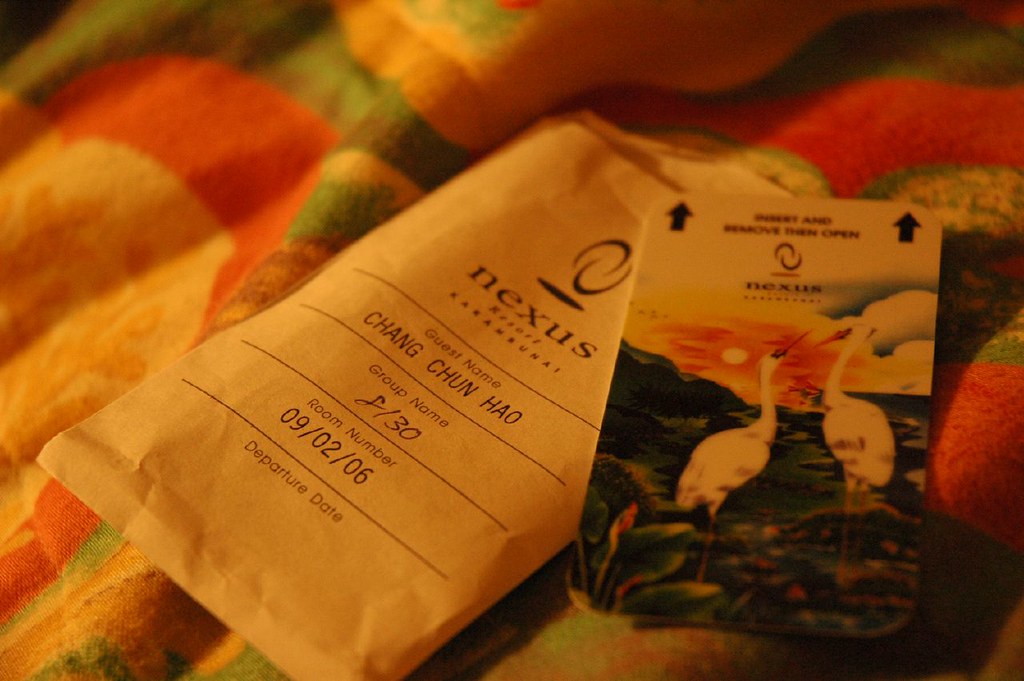The image showcases a colorful hotel room key card and the light lemon-yellow paper envelope that holds it, both lying on a bedspread with green, red, and yellow hues. The key card, positioned on the right, features an artistic rendering of two white birds, possibly herons or storks, with long beaks and black markings around their eyes. The background of the card is impressionistic, depicting a hillside with leafy vegetation, a setting red sun, and clouds. At the top of the card, "NEXUS" is printed in black letters above two arrows indicating the insertion direction. To the left, the partially visible envelope also reads "NEXUS," below which it lists the guest name "Chang Chun Hao," the group name "8130," the room number "8130," and the departure date "09/02/06." The vivid colors and detailed elements of the bedspread provide a harmonious backdrop for the key card and its envelope.